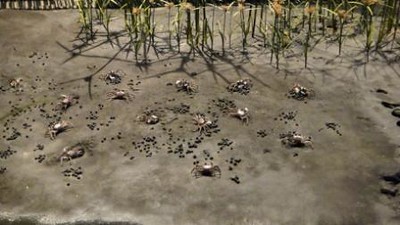The image captures a group of small crabs scurrying across a beach with light brown, sandy terrain. The sand appears uneven, with some damp patches suggesting recent wetness. Scattered darker brown debris dot the sand, possibly organic matter. The crabs create subtle indentations as they move, and while their exact size is unclear due to the distant and somewhat blurry quality of the photo, their essence is visible. In the background, there are sparse plants resembling corn stalks or reeds, displaying green stems that fade to tan at the top. Toward the image's edge, a faint line of stones is visible, and additional indistinct elements in the background hint at more distant features.